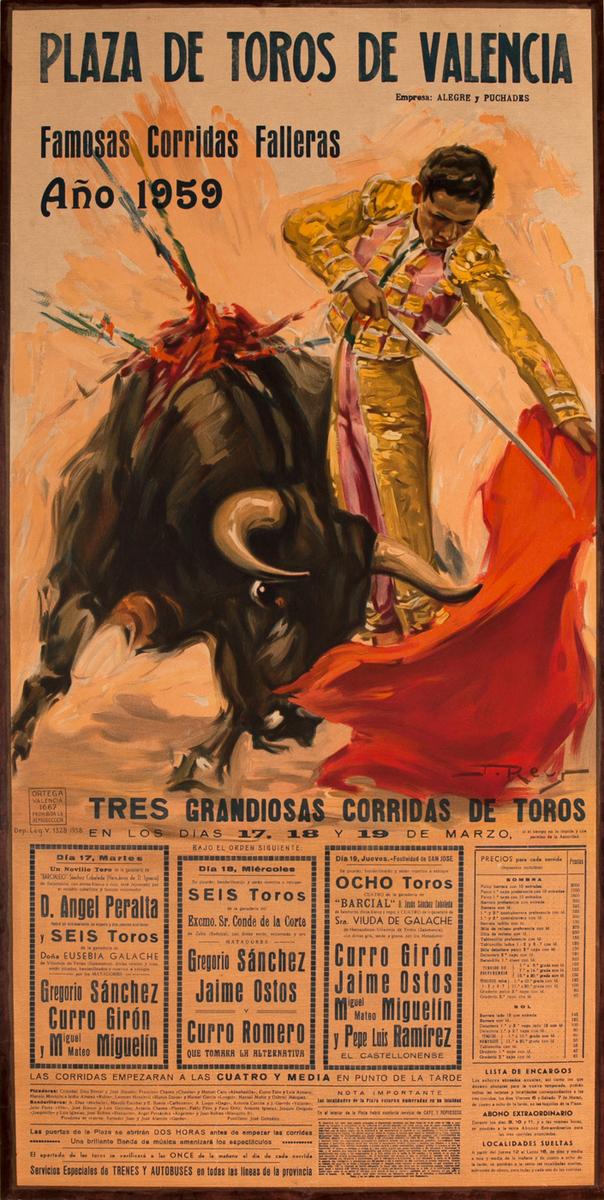This detailed poster from 1959 advertises a bullfight at the Plaza de Toros de Valencia. Predominantly orange, black, and white, the poster almost resembles newsprint. At the top, it reads "Plaza de Toros de Valencia" and mentions "Famosas Corridas Ferreiras" along with the year "1959." The central image is a dramatic painting featuring a matador in a yellow suit striking a poised stance, showcasing a red cape in one hand and a sword in the other. The black bull, with large horns and swords embedded in its back, aggressively charges at the red cape, embodying the intense and brutal nature of the spectacle. Further down, the poster details the grand event, stretching over two days, March 17th, 18th, and 19th, capturing the traditional bullfighting fervor of the era.